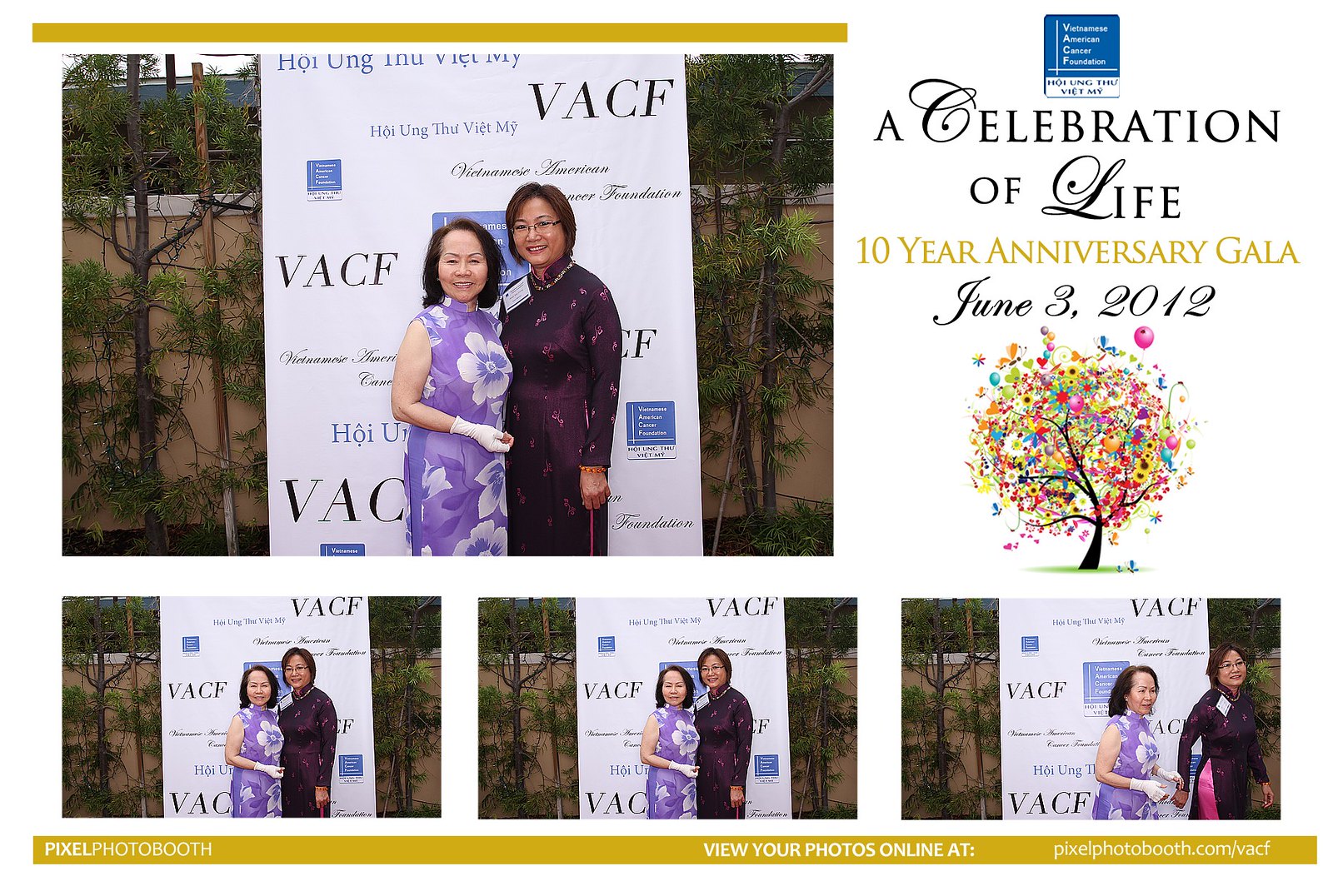The image showcases a collage of photographs from a "Celebration of Life, 10 Year Anniversary Gala" held on June 3rd, 2012. Central to the collage are multiple images of two mid-to-late 50s women, dressed in traditional Vietnamese clothing in purplish hues, posing in front of a sign that repeatedly displays "VACF" along with other Vietnamese text in cursive, mentioning something about a Vietnamese American foundation. Behind them, a backdrop reveals trees and a building. Notably, the top left of the collage features an illustration of a tree with rainbow-colored leaves and balloons against a grassy setting. Below these images, a golden banner directs viewers to "view your photos online at pixelphotobooth.com/BACF." The collage is vibrant with colors including yellow, green, brown, white, blue, purple, and pink, and appears to be an advertisement highlighting the gala event and its photographed moments.